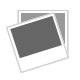This photograph depicts an antique, dark jade green wooden table, which shows signs of wear with several scuffs, positioned against a white wall. On top of the table sits an intricate wine bottle holder. The holder features an ornate design, beginning with a circular metal piece that threads through the top of the wine bottle. This metal piece connects to a stylized component resembling an elephant's head, complete with a trunk-like extension and ear-like features, likely made of pewter or a similar material. This decorative element links to an arched wooden arm, wrapped with twine, which curves downward toward the table, transitioning into a sleigh-like cradle that supports the body of the wine bottle. The base of the holder includes two leaf-like protrusions for added support. The entire structure, with its combination of metal and wood, creates an elegant yet rustic appearance, enhancing the antique charm of the table it rests upon.